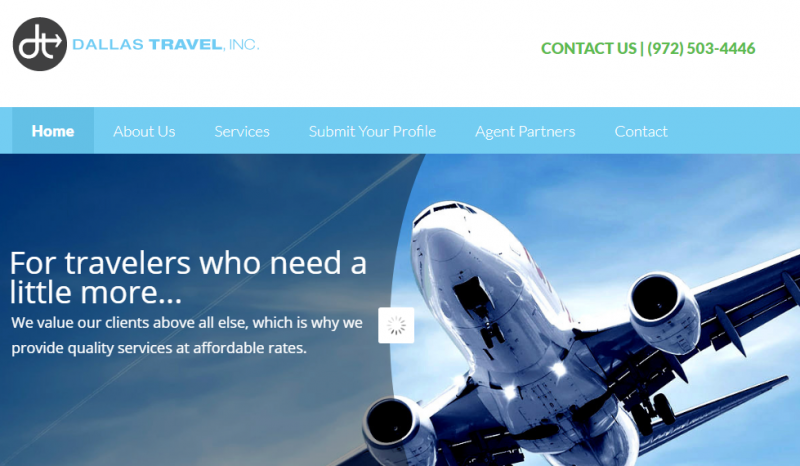Detailed Caption:

The image is a screenshot of the homepage of Dallas Travel, Inc., a professional travel services website. The logo, positioned on the top left corner, consists of the initials "DT" followed by "Dallas Travel, Inc." in bold blue lettering, with "Travel" notably emphasized. On the top right side, "Contact us at 972-503-446" is displayed in green, adding a pop of color to draw attention to their contact information.

The navigation menu at the top includes sections for Home, About Us, Services, Submit Your Profile, Agent Partners, and Contact, with the Home section currently selected. Below the navigation bar, there is a welcoming message that reads, "For travelers who need a little more, we value our clients above all else, which is why we provide quality services at affordable rates."

The center of the page features a dynamic loading icon next to the welcoming text, indicating some interactive or dynamic content on the page. The most striking element under this is a large, prominent image of an airplane taking off, which covers a significant portion of the screen, reinforcing the travel theme of the website.

The overall layout is clean and professional, utilizing a blue and white color scheme that conveys trust and reliability. The design is user-friendly, with accessible and easily readable navigation. The green contact information stands out against this color palette, ensuring it is easily noticeable.